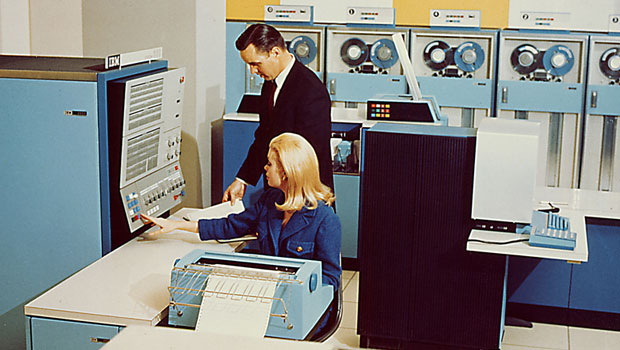The photograph, likely from the 1950s or 1960s, captures a computer room filled with large, bulky mainframe computers reminiscent of early IBM technology. A woman with sleek blonde hair, dressed in a blue suit, is seated at a desk operating an electric typewriter or a computer keyboard. To her right, she is pressing a button on a large rectangular machine with a metal screen and numerous buttons. Beside her, a man in a business suit leans over the table, examining some papers. The backdrop features multiple towering machines, including ones with circular reels at the top and bands of silver and white below, suggesting the use of magnetic tape storage. The setting exudes an atmosphere of an office or scientific establishment, with a vintage feel characterized by the fashion and technology of the era.